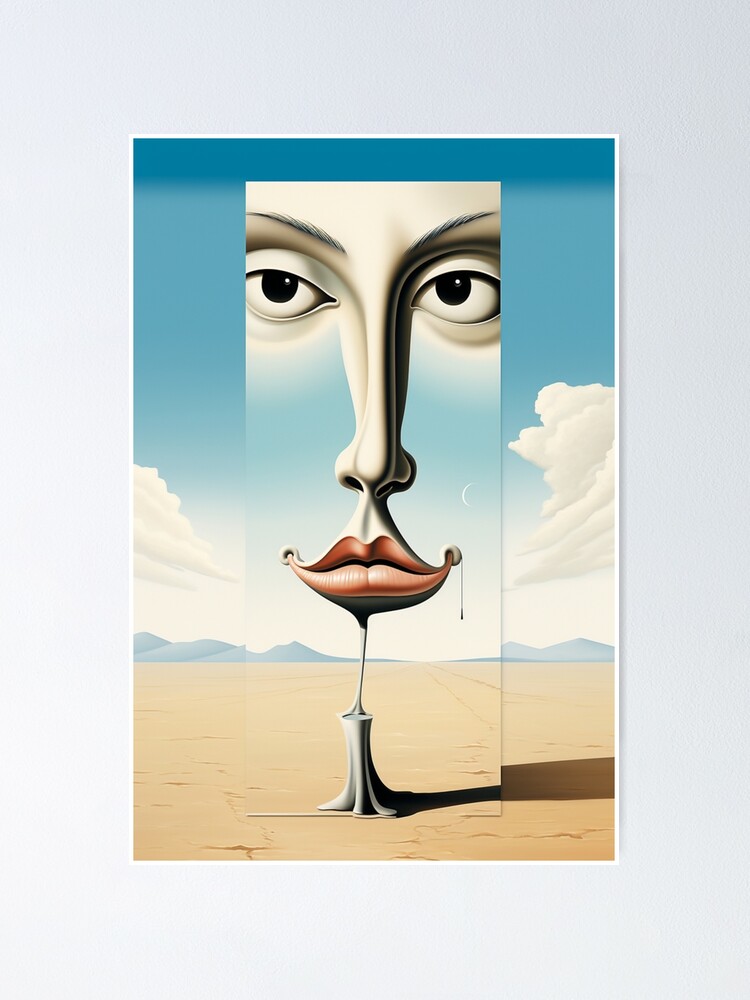This modern art piece presents a captivating surrealist scene that merges elements of a desert landscape with the features of a human face. Set against the stark expanse of tan sand in the middle of a desolate desert, a striking image emerges from the base of a gray tree trunk. The gray tree trunk transitions into a white spindle that supports an ethereal painting seamlessly integrated into the overall artwork. The painting prominently features a woman's face, characterized by half-lidded dark eyes, a long, narrow nose, and voluptuous lips with the top lip showcasing a deeper red hue than the bottom.

The sky above is a vibrant, intense blue, streaked with a few white clouds, and the distant horizon reveals gray-blue mountains, adding depth to the scene. The desert surrounding the central image is vast and unbroken, depicted in light brown hues. The overall scene is framed by a thin white border, enhancing its three-dimensional feel and adding to the surreal quality of the composition. The detailed rendering of shadows indicates a bright, sunny day, emphasizing the artist's masterful use of light and shadow to create a sense of realism within the surreal.

This piece, reminiscent of Salvador Dali's works, blends the realistic with the fantastical, creating a mesmerizing and unique visual experience where the transparent facial features seemingly float in the desert sky, capturing the viewer's gaze and evoking a sense of mystery and wonder.